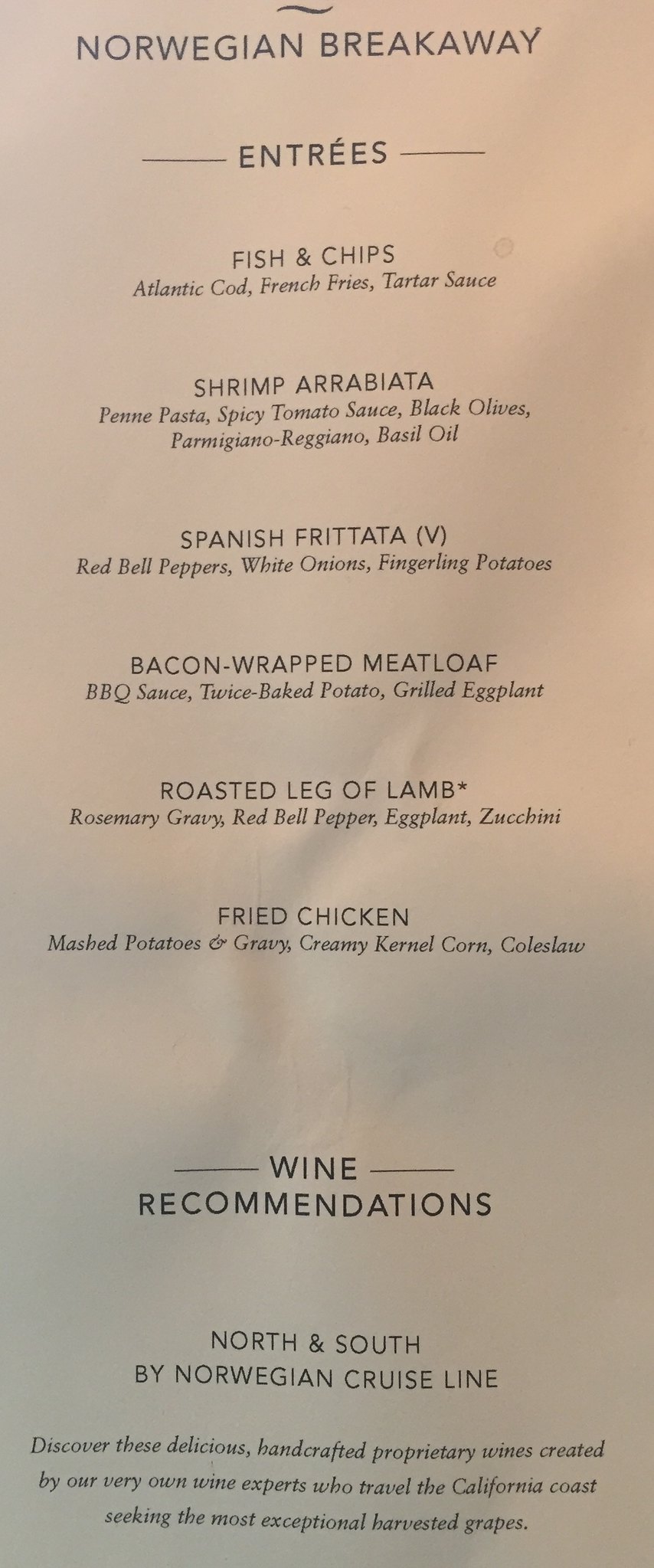This vertical image, significantly taller than it is wide, depicts a menu from Norwegian Cruise Lines. The menu is primarily a dark tan with a dark brown or black print, offering a visually striking contrast. Highlighted at the top of the menu is the name of the ship, Norwegian Breakaway. 

The detailed list of entrées includes:

- **Fish and Chips**: Classic pub fare with a crispy exterior and tender fish inside.
- **Shrimp Arabica**: Juicy shrimp seasoned with aromatic spices.
- **Spanish Frittata**: A hearty egg dish filled with various flavorful ingredients.
- **Bacon-Wrapped Meatloaf**: Rich meatloaf encased in crispy bacon.
- **Roasted Leg of Lamb**: Succulent lamb roasted to perfection.
- **Fried Chicken**: Crispy, golden-brown pieces of chicken.

Each entrée is accompanied by descriptions of the sides that complement the dishes, although specific details of these sides are not provided in the caption.

The bottom third of the menu is dedicated to wine recommendations under the banner "North and South by Norwegian Cruise Line." It features a promotional statement which reads: "Discover these delicious handcrafted proprietary wines created by our very own wine experts who travel the California coast seeking the most exceptional harvested grapes."

Notably, there are no prices listed on the menu, suggesting that these sumptuous meal options are likely included in the cruise fare, offering guests a taste of luxury as part of their overall experience on the Norwegian Breakaway.